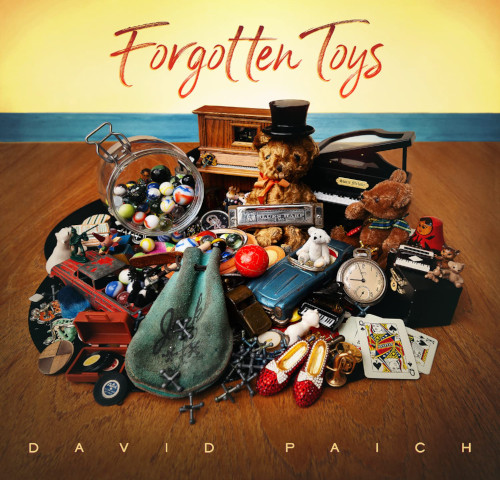The image appears to be the cover of a book or album titled "Forgotten Toys," displayed prominently in a faded red script font on a yellow background at the top. Below, the scene transitions into what resembles a sky with a blue ocean-like expanse. The setting is a cluttered wooden floor, strewn with a diverse array of toys and nostalgic items, seemingly haphazardly piled together. 

At the center of the collection is a distorted teddy bear with an orange bow and a black top hat, missing one eye, with a harmonica placed across its lap. Surrounding the bear are ruby red slippers with white bows, a clear glass jar filled with colorful marbles, silver jacks, and playing cards. Also visible are various other objects including upright and grand pianos, balls, watches, shoes, tires, a clock, ballerina shoes, and possibly a Funko Pop and a little record player. The detailed mishmash of items evokes memories of childhood playthings, now abandoned and forgotten.

Near the bottom, in a light yellow font, is the author’s or artist’s name, David Paich, solidifying the nostalgic and somewhat melancholic theme of the assembled memorabilia.